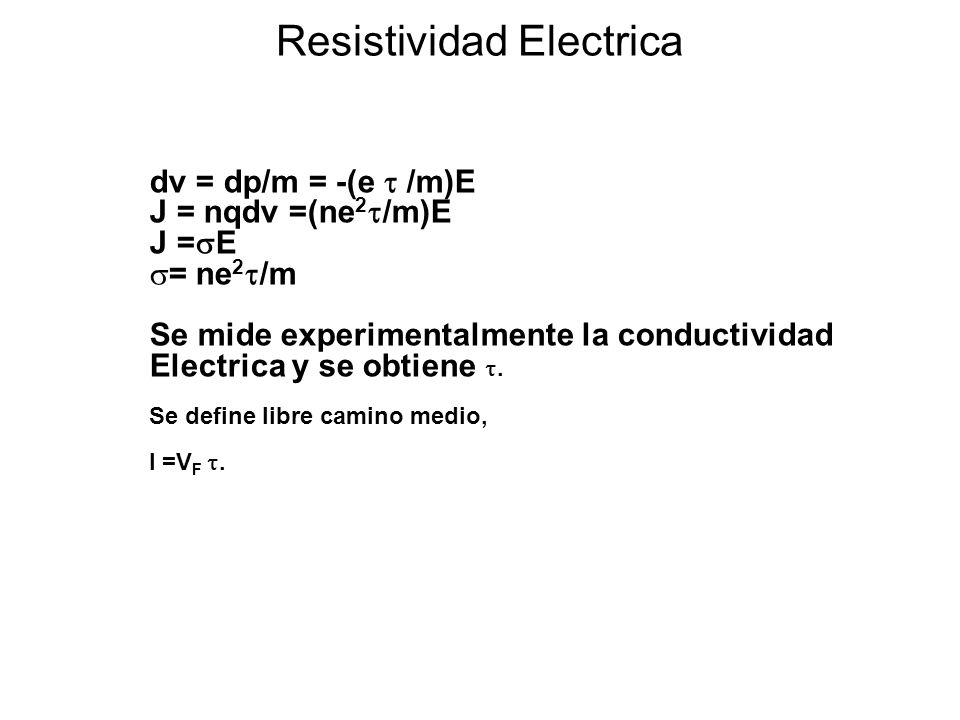The image features centered black text on a white background with the title "Resistividad Eléctrica" prominently displayed at the top. Below the title, there are several mathematical formulas written in black font, each stacked one above the other. The first formula reads "dV = dP / m = - (e / m) * E." The second formula states "J = nQ dV = (ne² / m) * E," while the third line repeats with "J = a circle with a line through it E = ne² / m." The text also includes some Spanish sentences such as "Si mire experimental conductividad eléctrica y si obtener," followed by "si define a libre camino medio." The entire image comprises a total of nine lines, culminating in the simplicity of black lettering on a white background, focusing distinctly on the mathematical expressions and their components.